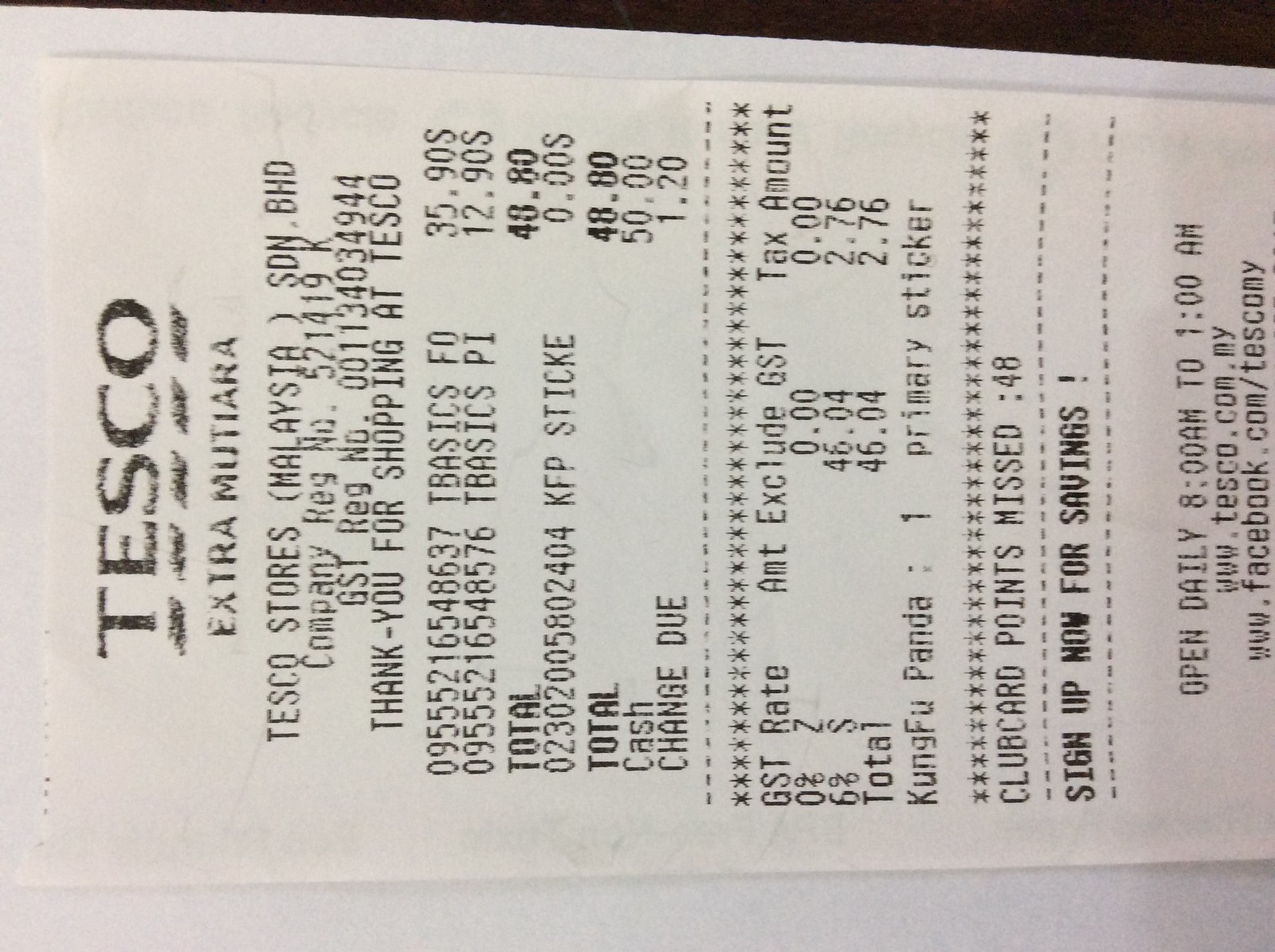This is a photograph of a Tesco receipt printed on white thermal paper with black text. The receipt is slightly obscured by a bit of black in the top right corner, and there is a small white area at the bottom. Prominently displayed in the middle of the receipt are the bold black letters "Tesco," underlined by a square. Below this, it reads "Extra Mutaria."

The receipt identifies the store as located in Malaysia, featuring a company registration number of 521-419-K and a GST registration number. Following this, the message "Thank you for shopping at Tesco" is printed.

The receipt details the purchases made, including items listed as T-Basics Fo and T-Basics Pi, with respective costs of $35.90 and $12.90, leading to a total of $48.80. The shopper paid $50 in cash and received $1.20 as change.

Additional information includes the text "Kung Fu Panda 1, primary sticker" and a mention of "Club card points missed: 48," encouraging customers to sign up for savings.